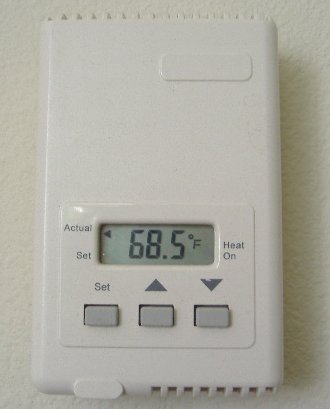The image prominently features a thermostat against a beige-colored wall, with the thermostat itself in an off-white, eggshell hue that blends with the wall. The device has a minimalistic design, with visible heat sinks located at the top and bottom. On the upper right corner, there is a small, embossed plastic indicator. 

The control panel includes three raised gray buttons: "SET," "UP," and "DOWN," located along the bottom edge. The digital display shows a temperature of 68.5°F. On the left side of the display, the terms "ACTUAL" and "SET" are noted, with an arrow pointing to "ACTUAL," indicating that 68.5°F is the current room temperature. The right side of the display features the label "HEAT ON," but it is not activated, suggesting the heating system is off.

The image is illuminated from the left side, creating a soft shadow that extends slightly to the right behind the thermostat. The shadow's presence subtly enhances the depth and realism of the scene. The overall composition emphasizes the simplicity and functionality of the thermostat within its setting.